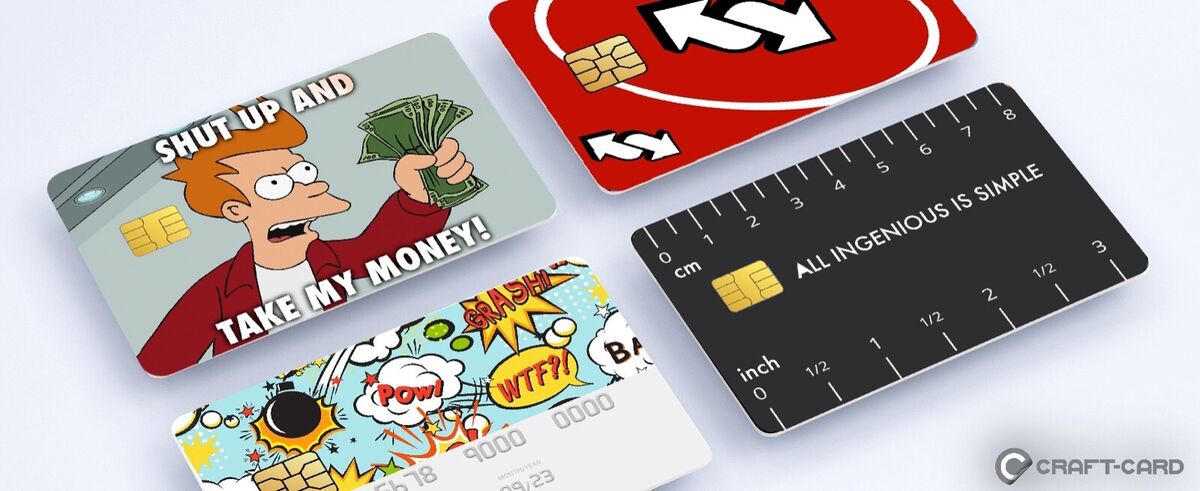The image showcases four customized credit card designs floating above a white surface, bearing the Craft Dash Card logo, a 'C' in a semi-circle, in the bottom right. Each card is distinct and features playful, graphic elements. The top left card displays Fry from Futurama with the phrase "Shut Up and Take My Money!" Fry holds cash, wearing a red jacket and white shirt, with an embedded gold chip to the left side. Adjacent to it, the top right card has a bold red background with a white circle and yellow UNO reverse arrows, accompanied by another gold chip. The bottom left card features a comic-style explosion with a black bomb and starburst that reads "POW" and "CRASH," followed by "WTF?!" in a yellow speech bubble, with numerical details below mimicking credit card digits. The bottom right card is sleek black with the phrase "All Ingenious is Simple" in the center, resembling a ruler with measurements in centimeters and inches along its edges and another gold chip near the text. The overall design cleverly integrates amusing and dynamic visual elements typical of meme culture within the framework of credit card aesthetics.